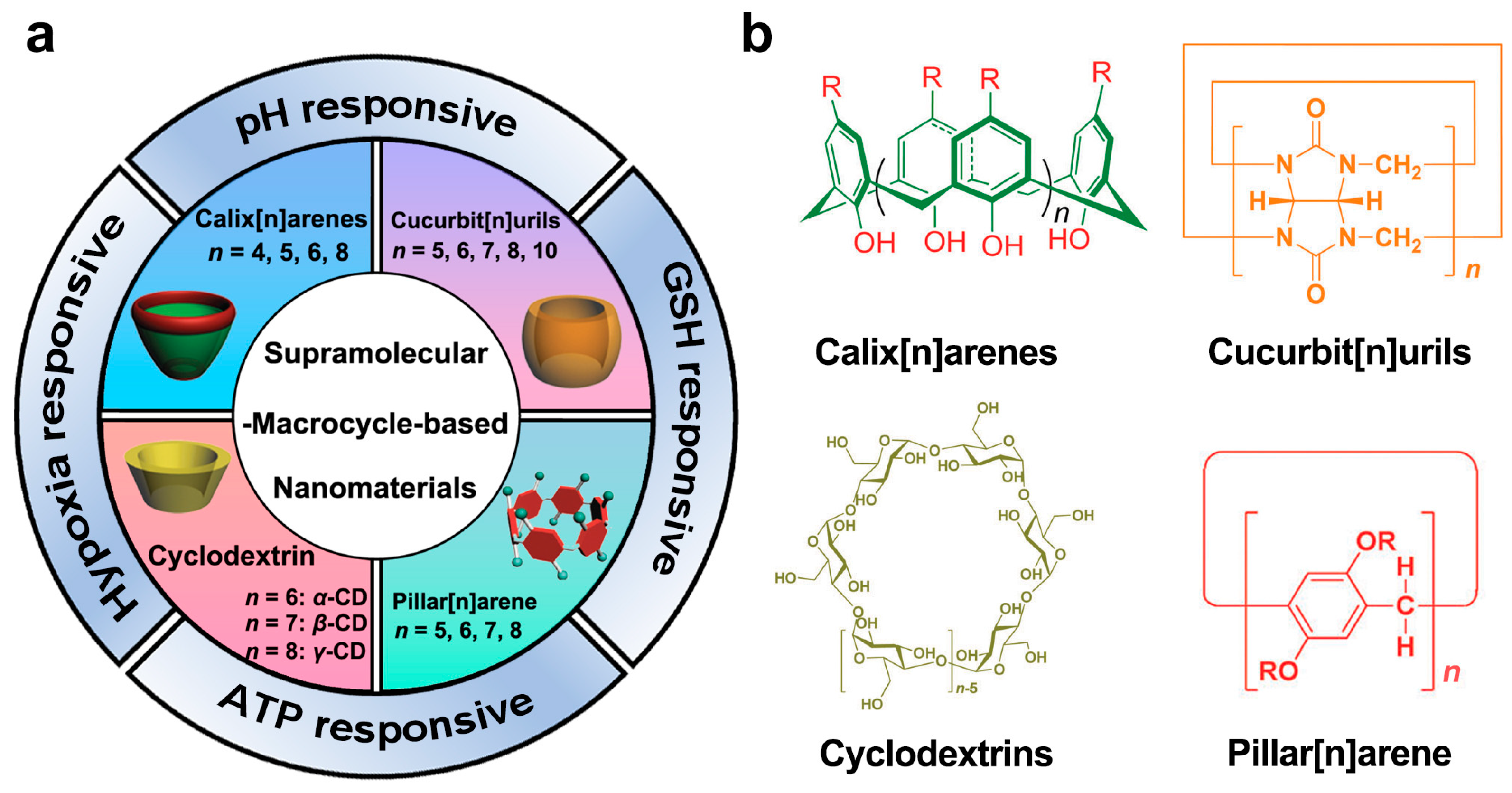This informational image is divided into two sections, labeled A and B, against a white background. Section A on the left features a circular diagram resembling a pie chart, divided into four color-coded quadrants: blue, purple, pink, and aqua. Each quadrant represents responsiveness levels—pH responsive, GSH responsive, ATP responsive, and hypoxia responsive—written in black text. The center of this diagram contains the terms "supramolecular," "macrocycle-based," and "nanomaterials." Surrounding the circle, the quadrants correspond to four categories: calixarene, cucurbituril, pillararene, and cyclodextrin.

On the right side, section B displays the molecular structures of these four categories. These structures are depicted in different colors: green for calixarene, orange for cucurbituril, brown for pillararene, and red for cyclodextrin. Beneath each molecular diagram, the respective name is clearly labeled in black text. The image effectively conveys the detailed chemical information and hierarchical responsiveness represented through these vibrant diagrams.